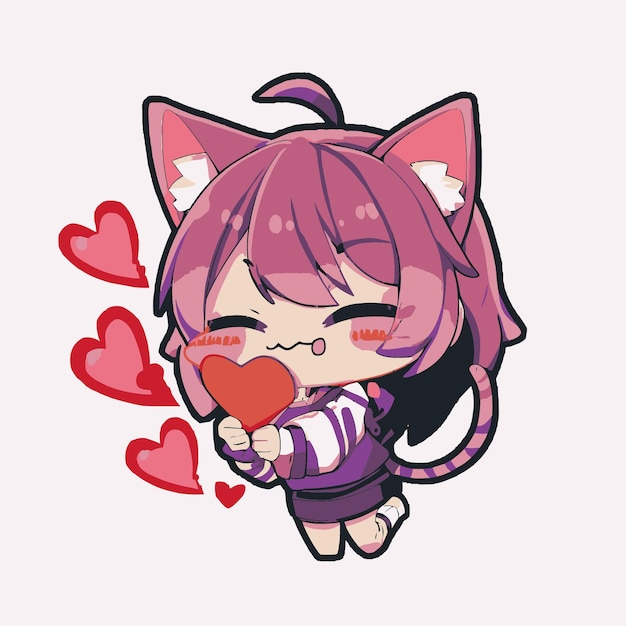This vibrant square-format anime illustration depicts a young girl with large, purplish-pink hair styled in a ponytail, adorned with cat-like pink ears. Her eyes are squinty, and her tongue playfully sticks out, emphasizing her joyous expression. She wears a sporty, purple school uniform complemented by white socks. In her hands, she holds a red Valentine heart, a gift that has evidently thrilled her. Surrounding her, three floating hearts in shades of red and pink visually express her elation. Her purple and pink checkered tail adds an extra layer of cuteness to the image, with one part standing up and another playfully kicking behind her. The illustration expertly conveys a sense of kawaii charm and excitement, encapsulating the heartfelt moment of receiving a Valentine.